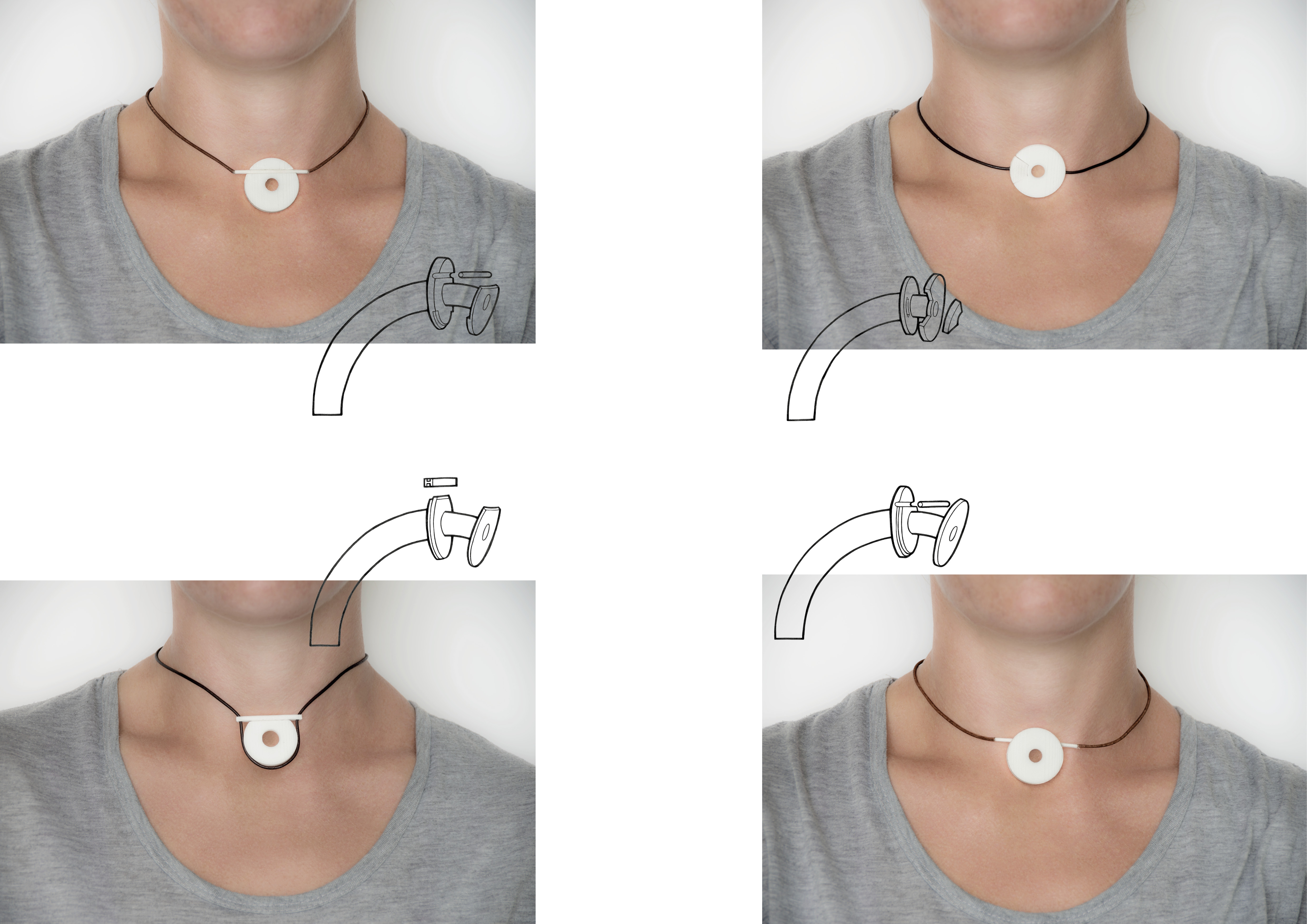The image is a grid of four photographs showcasing a device designed for individuals with tracheotomies. Each photograph focuses on the neck, collarbone, and shoulders of a woman wearing the same gray shirt with a low neckline. The device, which resembles a necklace, consists of a single black band and a white washer-like element at its center. In each image, different methods of attaching and arranging the necklace around the neck are illustrated. The top left photo displays a diagram showing a pin inserted through the top of the back plate, with the front plate clipping over it to suspend the pendant. The top right, bottom left, and bottom right photos each feature distinct diagrams illustrating alternative configurations for suspending the pendant on the black band. These images collectively highlight various ways to wear and customize the necklace, emphasizing its adaptability and functionality for covering a tracheostomy tube.